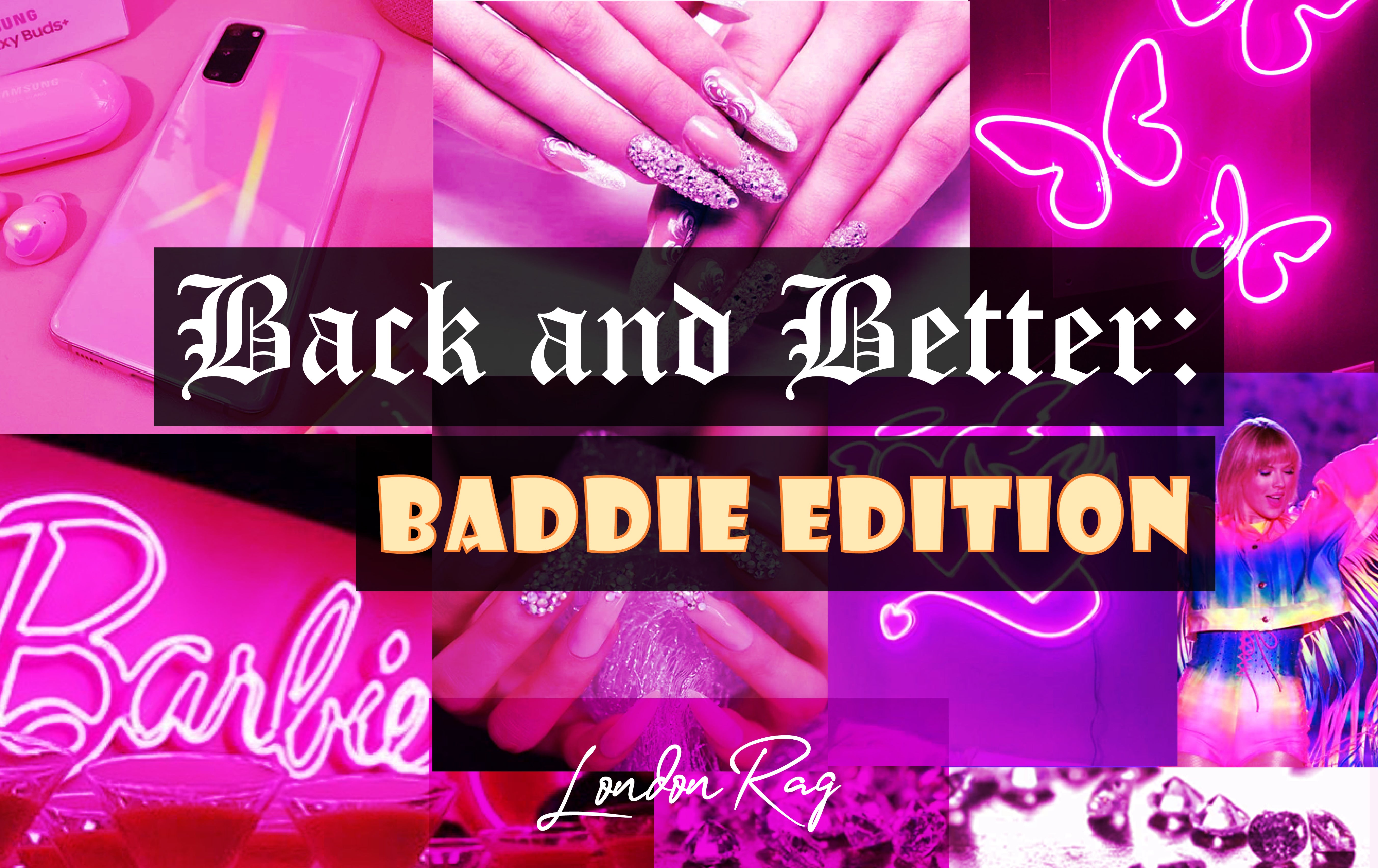The image is a vibrant, pink-themed advertisement. Dominating the center is bold typography on a black background with white print, reading "Back and Better," followed by the phrase "Baddie Edition" in yellow lettering. The background comprises a collage of images: a pink cell phone, a girl with long, sparkly pink fingernails, and a scene with white neon butterflies set against a pink backdrop. Additional visuals include a neon sign spelling "Barbie," pink fingernails, and a squiggly neon heart. There is also a girl, possibly resembling Taylor Swift, in a blue outfit holding fuzzy blue items. Scattered in the layout are pink and purple sapphire-like jewels. At the bottom, the cursive text "London Rag" serves as a signature element. The collage is arranged in a grid pattern with nine distinct sections, underscoring the pink and purple hues prevalent throughout.